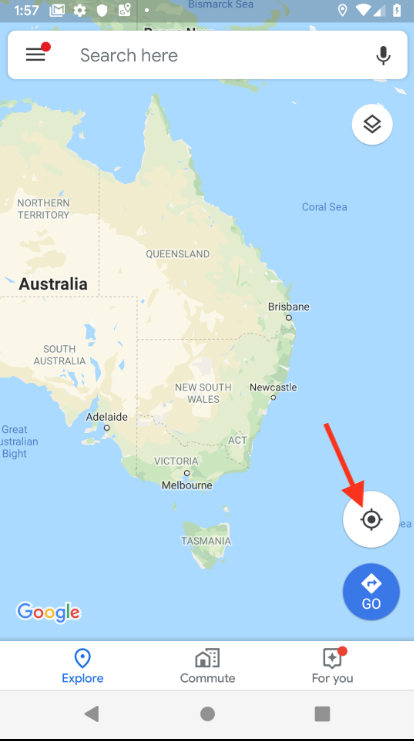This is a detailed screenshot from a tablet or smartphone, evident from the semi-transparent status bar at the top, alongside icons typically found on mobile devices. 

- **Top Left Corner**: The time displayed is 11:57, without an AM or PM designation, suggesting it could be in military time.
- **Top Bar Icons**: Features from left to right include:
  1. **Google Logo** surrounded by multiple small squares, hinting at multiple Gmail messages.
  2. **Gear Icon** for settings.
  3. A **Shield Icon**, possibly linked to security settings.
  4. **Map Icon** with a 'G' symbol, pinpoint, and additional details likely related to Google Maps.
  5. A **white period** symbol.
- **Center of the Top Bar**: In bold black text within a rectangle is "Vismarc", which stands for "Bismarck" but notably spelled as "V-I-S-M-A-R-C-C".
- **Top Right Corner**: Shows a pin icon, a complete Wi-Fi signal, mobile signal strength rated just below two-thirds, and a fully charged battery with a lightning bolt indicating it is charging.

**Search Bar**:
- Left side: Three lines which suggest additional settings. A red circle here indicates a notification.
- Text inside: “Search here”.
- Right side: A Google Assistant microphone icon, facilitating voice search.

**Map Display**:
- **Central Feature**: A map of Australia, though ‘Australia’ is misspelled as 'A-U-S-T-R-A-I-L-A'.
- Red arrow pointing to a gray circle with a black, four-lined circle inside, possibly for pinning locations.
- A blue arrow inside a dark blue circle with a diamond icon saying “Go” indicates starting navigation.

**Additional Icons**:
- Below the search bar: A gray circle featuring a black outline of another square, likely used for uploading.

**Bottom Bar**:
- **"Explore"** section chosen, symbolized by a pin icon on the gray bottom bezel.
- **"Commute"** section with icons of a house and a skyscraper.
- **"For You"** section: Illustrated by a bookmark with a star and highlighted by a red circle for notifications.

**Navigation Buttons**:
- Located in a darker gray bezel at the phone’s bottom: A back arrow, a home circle, and a multitask square for switching between apps or going home.

This thorough detail encapsulates various functionalities and notifications visible on the device's screen, emphasizing its design and user interface.